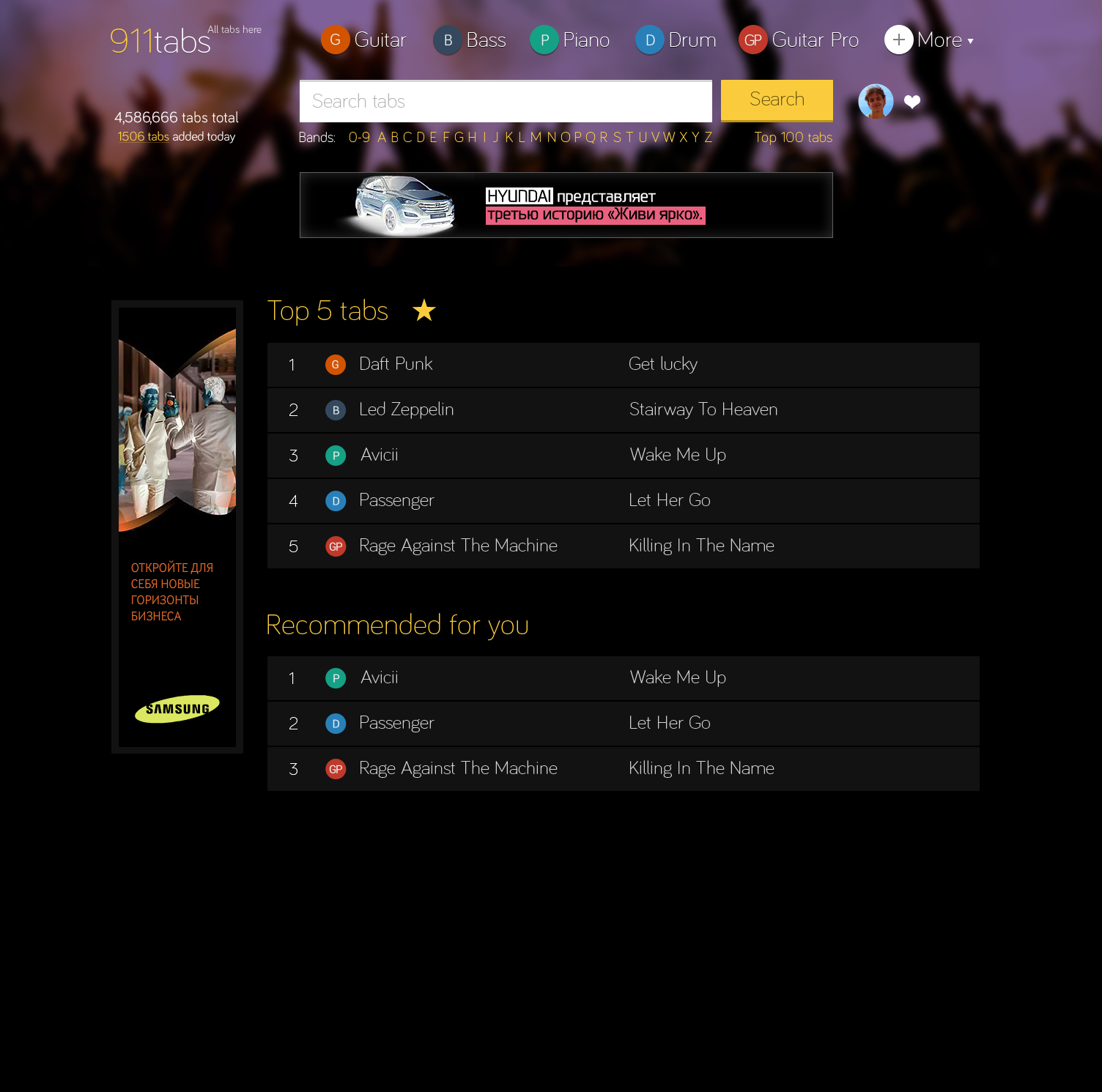The image depicts a sleek, music-dedicated website with a predominantly black background that transitions to purple at the top, where black silhouettes add a layer of depth. In the top-left corner, the text reads "911 Tabs," and to its right are five categorized tabs: Guitar, Bass, Piano, Drum, and Guitar Pro. Next to these tabs is a profile icon. 

Beneath this, a white search bar is situated with a yellow "Search" button adjacent to it, followed by a blue headphones icon. Directly below the search bar is an advertisement block. 

The first main content section is titled "Top 5 Tabs," with a list of tabs ranked from one to five. Each entry features the artist's name on the left and the track name on the right, all placed against a dark gray backdrop.

Following this is a "Recommended for You" section, highlighted in yellow text. Here, the artist names are positioned to the left of the track names, maintaining the same aesthetic consistency.

At the very bottom left of the image is a prominent yellow Samsung logo, completing the webpage's design.